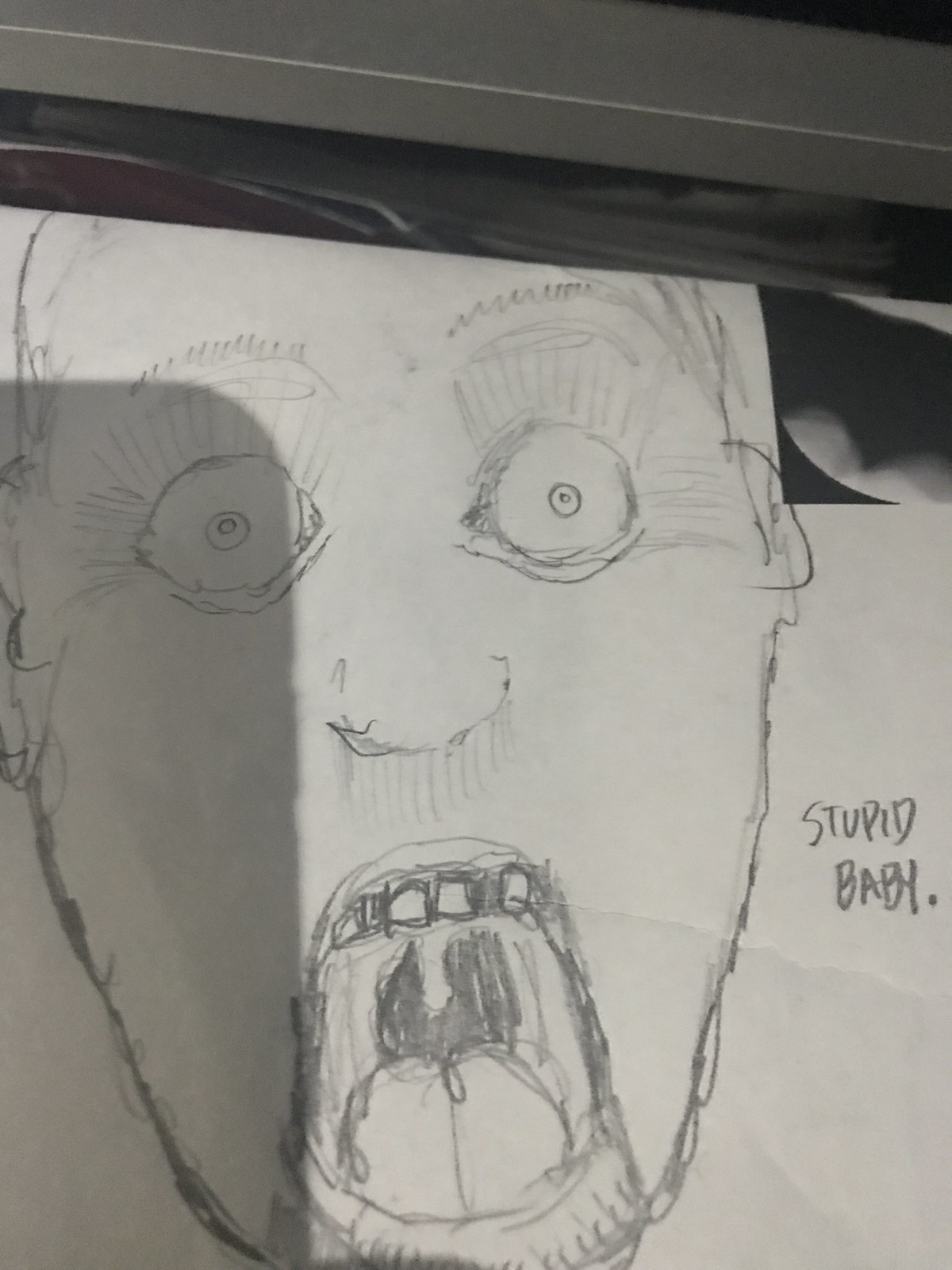This image features a close-up photograph of a pencil sketch depicting a man's head with an expression of extreme shock or terror. The face, apparently cut out from the surrounding paper, showcases wide, round eyes with very small irises and simple pencil-marked eyelashes and eyebrows, giving the appearance of lifted, alarmed eyebrows. The nose is a straightforward U-shape, and directly below it, pencil lines indicate depth. The man's mouth is wide open, revealing the top row of teeth, clearly drawn tonsils, and a tongue placed at the bottom of the mouth. The mouth's corners and the back of the throat are detailed with additional pencil scribbles, and the man appears to have a pencil-scribbled beard along the sides of his face. Above the sketched head, the photograph captures an unclear plastic bar, possibly the lid of a scanner. Notably, the right side of the drawing features the capitalized words "STUPID BABY," and there's a faint shadow of a smartphone on the left, indicating the photo was likely taken with a phone. The paper used appears to be a standard A4 sheet.